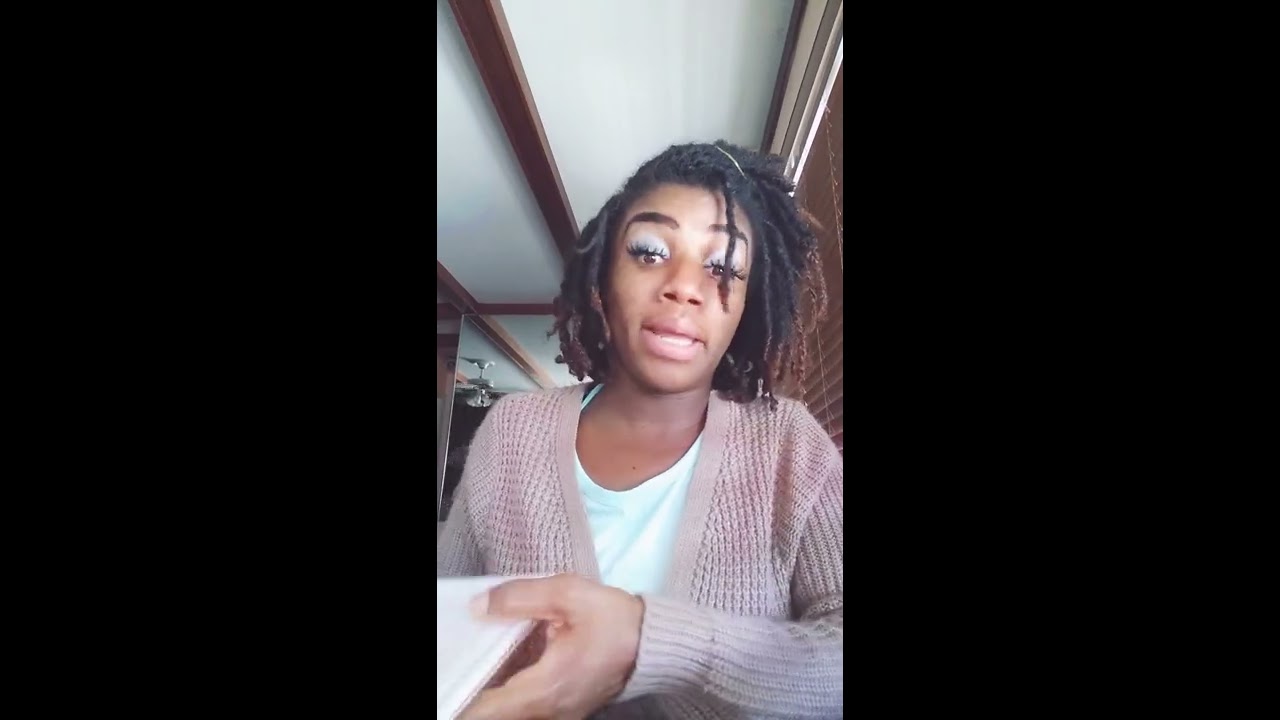In this wide rectangular image, a young black woman is depicted from the torso up, centered in a tall rectangular photo surrounded by black borders on both sides. She has short, curly black and brown dreadlocked hair that reaches her shoulders and features black eyebrows. Her dark skin contrasts with her bright, glittery blue eyeshadow and long eyelashes. She is in the middle of speaking, revealing the lower part of her teeth. The woman is wearing a grayish-pink, knitted, long-sleeve sweater vest over a white t-shirt. She is holding a white plate in her right hand, which extends towards the bottom left corner of the image. The background shows a room with a white ceiling adorned with long dark brown wooden panels and a window covered by brown horizontal blinds on her right. There is also a silver light fixture visible to the left in the background.